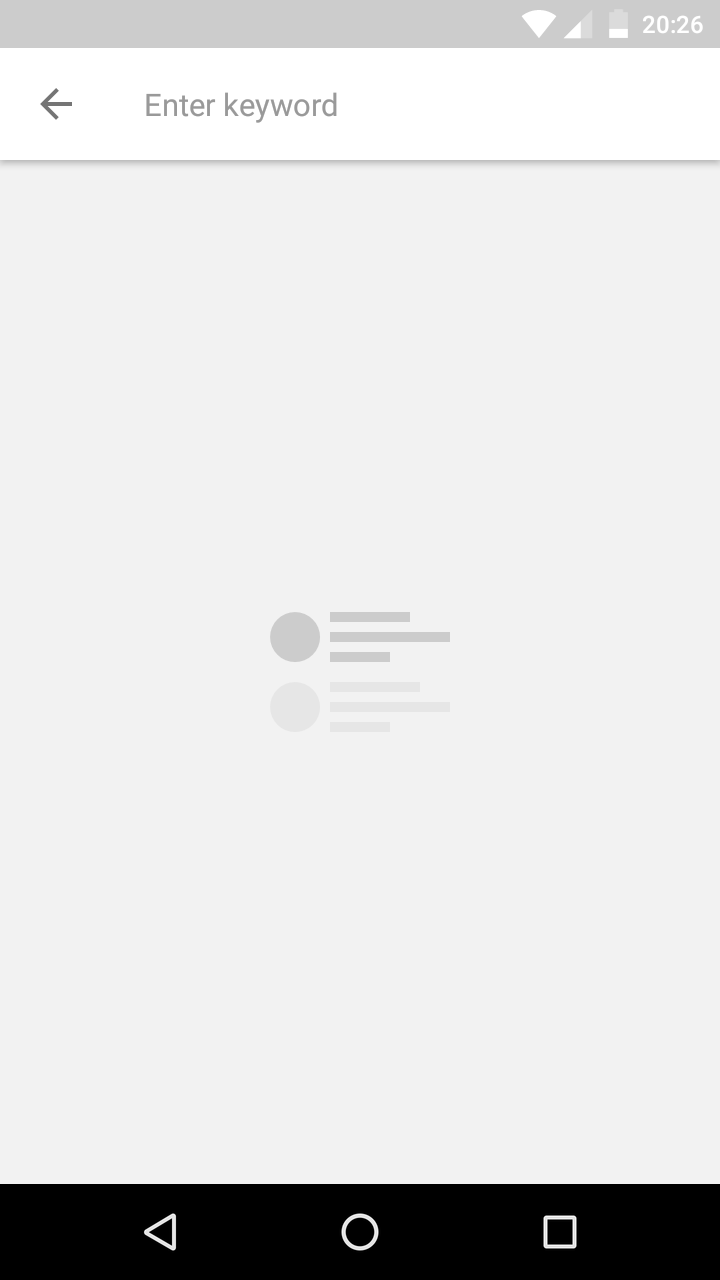A screenshot from a mobile device, possibly a prototype or placeholder, displays the standard interface elements. The top of the screen features the usual menu bar, indicating full Wi-Fi bars, a mobile signal strength of three bars, and a battery level below 50%. The time is shown as 20:26. Below the menu bar is the primary app interface which includes a back arrow on the left and a search bar with the placeholder text "Enter keyword," all set against a white background. A gray line divides this section from the main content area, which has a light gray background. This area appears mostly empty, possibly indicating a loading status, with two small circles and some lines that resemble indicators of a loading process. At the bottom of the screen, the typical navigation icons—back, circle (home), and square (recent apps)—are visible.